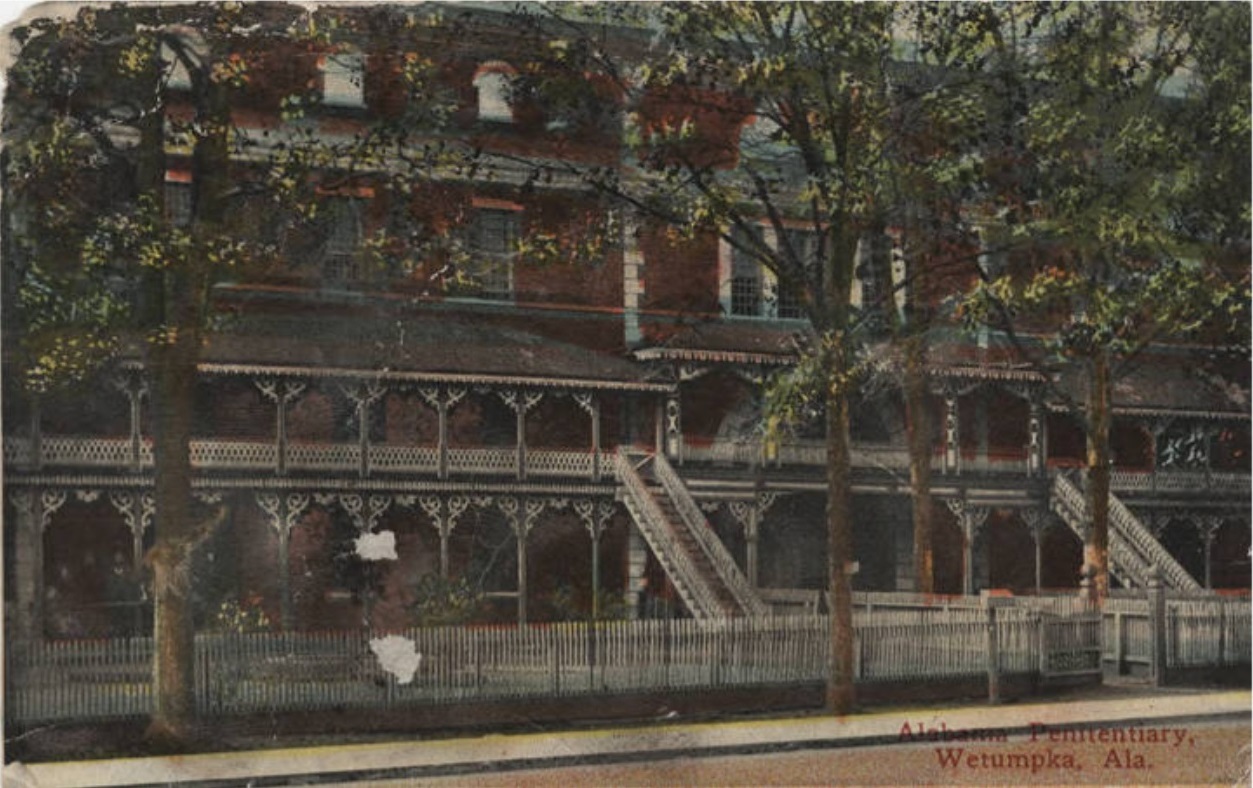This image depicts an artist's detailed painting of a large, red brick edifice labeled "Alabama Penitentiary, Wetumpka, Alabama" in red text at the bottom right corner. The imposing four-story structure features expansive wraparound balconies on the first and second floors, accentuated by white trellis banisters adorned with hanging flowers. Two prominent white staircases lead up to the second floor from the sidewalk, adding to the grandeur of the building. A neat white picket fence stretches across the lower part of the image, with an open gate and a mailbox near the entrance. Tall green-leaved trees line the sidewalk in front of the penitentiary, which is surrounded by carefully planted flowers, adding to the scene's tranquil yet striking composition.